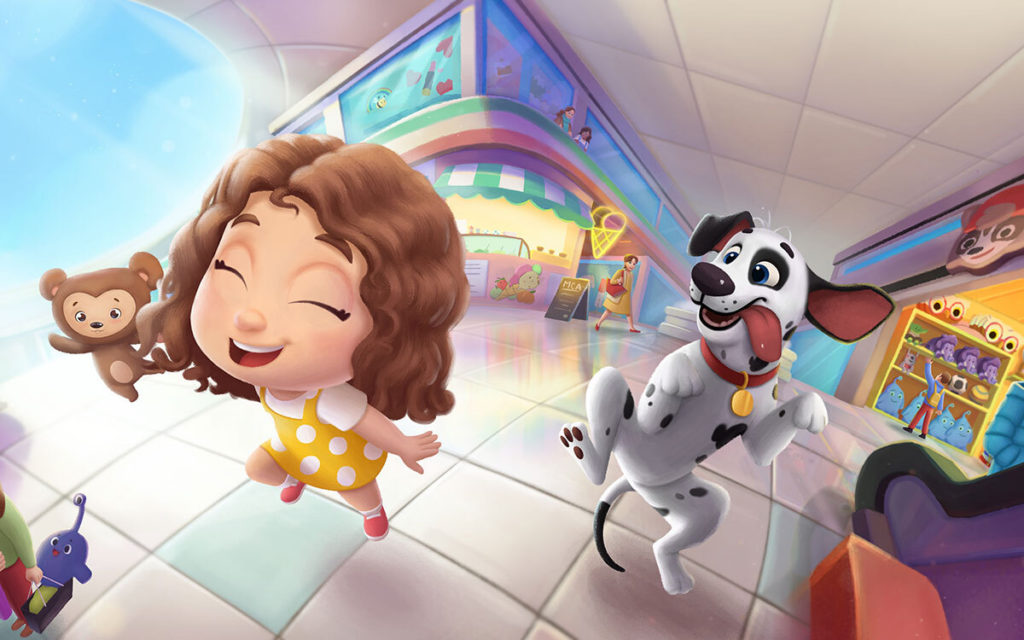In this computer-generated landscape-oriented image, a lively scene unfolds within a mall-like environment, featuring white tiled floors interspersed with a few teal tiles. Central to the image is a joyous little girl with light brown wavy hair, wearing a white dress adorned with yellow polka dots and red shoes. Her eyes are closed in happiness, and she appears to be jumping or skipping excitedly, all while holding a small stuffed monkey in her left hand. Accompanying her is a Dalmatian dog, also caught mid-jump, with its tongue playfully sticking out and sporting a red collar with a gold pendant.

To the far left, another child can be seen, dressed in a green top and red bottoms, carrying a black bag with a blue toy inside. The background reveals a bustling mall scene with a second level visible and multiple shops. Notably, there's an ice cream shop with a chalkboard sign and a person carrying a red bag walking past it. Nearby, there’s a toy store and what might be the bottom of an escalator peeking into the frame. The overall atmosphere is one of delight and vibrancy, capturing a joyful moment within this bustling indoor space.